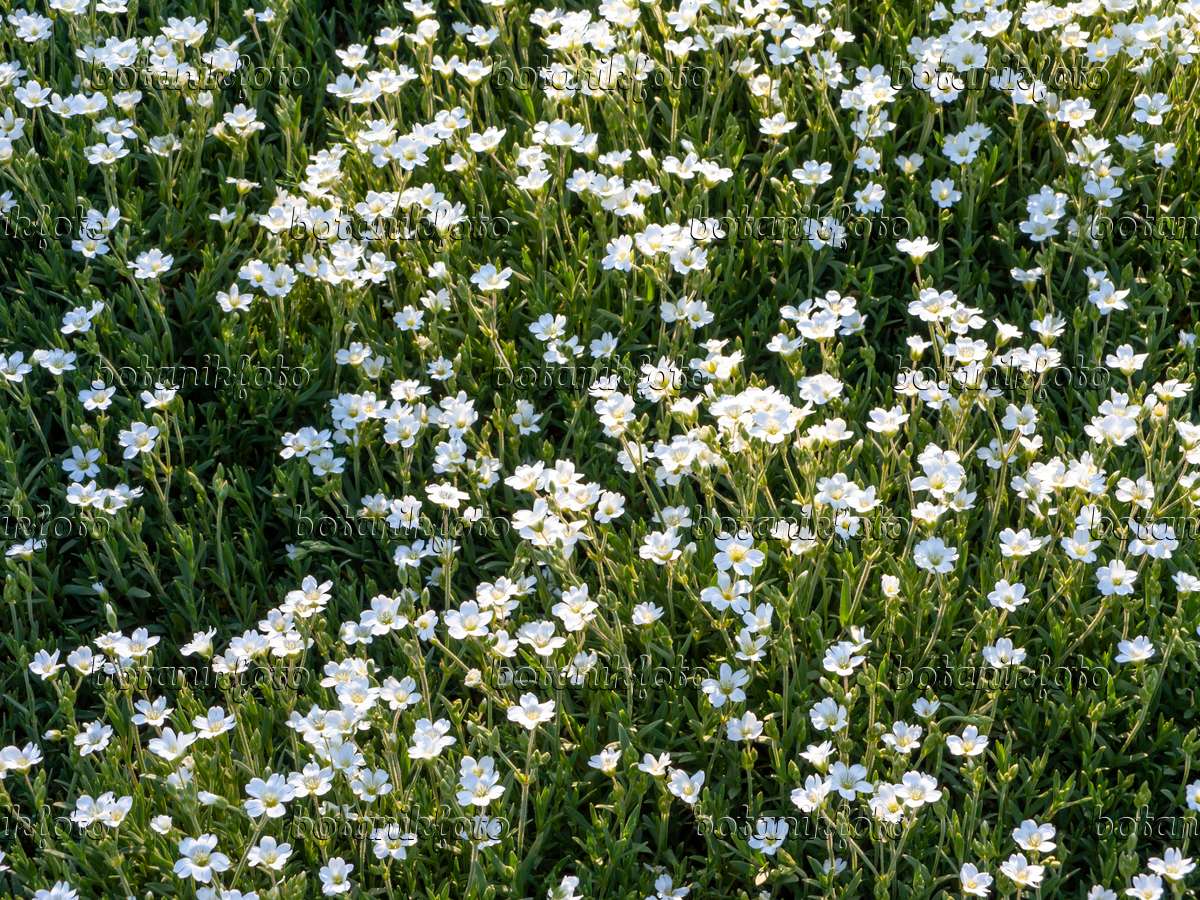This captivating photograph captures a vibrant display of a field densely packed with small white flowers, each boasting a modest yet elegant structure. The flowers have a cluster of tiny yellow stamens at the center, encircled by typically five delicate, oval-shaped petals that radiate upwards like spokes of a tiny wheel. Bathed in sunlight, these flowers stand straight and unwilted, exuding a soft, almost luminescent quality. The lush green foliage around them consists of narrow, elongated leaves, forming a dense, cushion-like undergrowth from which the flowers rise. It's a sunny day, and the scene invokes a serene sense of peacefulness, reminiscent of an untouched meadow. Amid the uniform sea of white and yellow, one can spot some dark hues between the flowers and budding shoots on the stems. The image is overlaid with a cursive watermark spelling "Botanik Foto" in horizontal lines, covering the photo entirely.